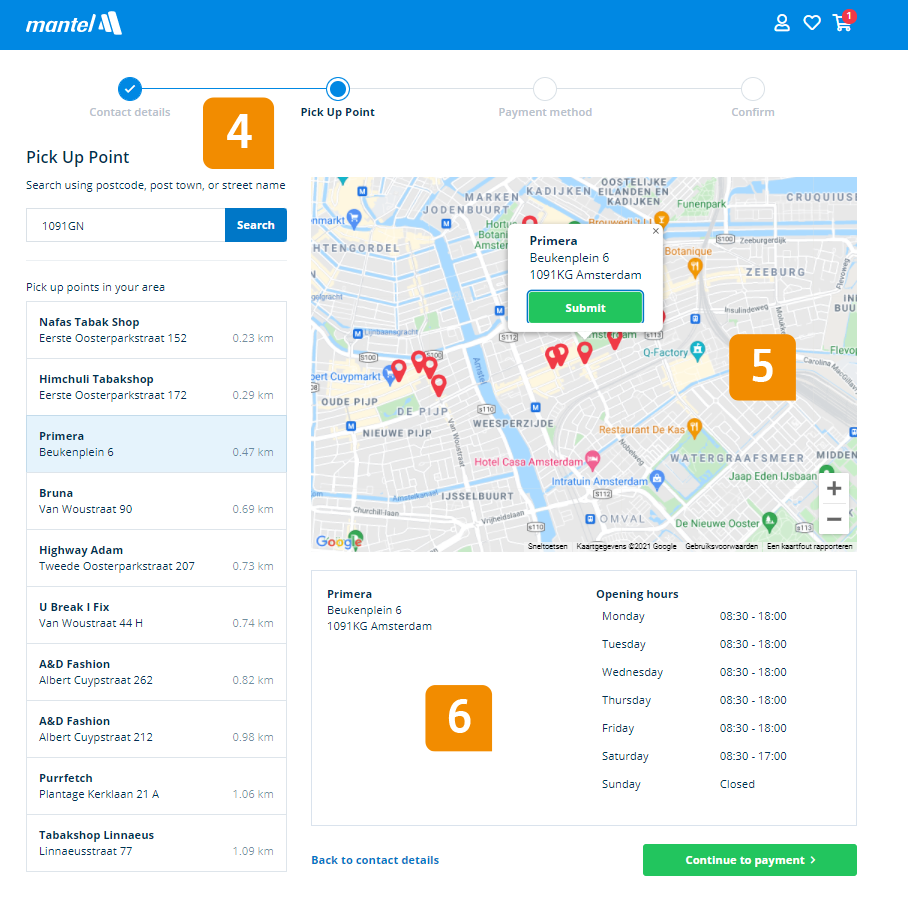A detailed digital interface displayed on the screen shows the scheduling process for a ride-sharing service named "Mantel." At the top of the page, the header indicates the service name along with a progress bar that highlights completed steps. The current steps, "Contact Information" and "Pickup Point," are marked in blue, signifying their completion. The subsequent steps to be completed are "Payment Method" and "Confirm."

Beneath the progress bar, the pickup point has been entered, though the exact location identifier isn't clear. The system automatically detects that the request is coming from Amsterdam and provides a list of nearby pickup locations. These options range in distance from 0.23 kilometers to 1.09 kilometers from the user's location, all within a reasonable walking distance.

The nearest pickup spot is labeled "Primera" and the address is listed as "Boekenplein 6, Amsterdam." Notably, the information appears to be in Dutch, hinting that the service caters to local users. Operating hours for each location are displayed in a 24-hour clock format.

At the bottom of the interface, a prominent "Continue to Payment" button encourages the user to proceed to the next step of selecting a payment method, ensuring a streamlined and guided process for scheduling their ride.